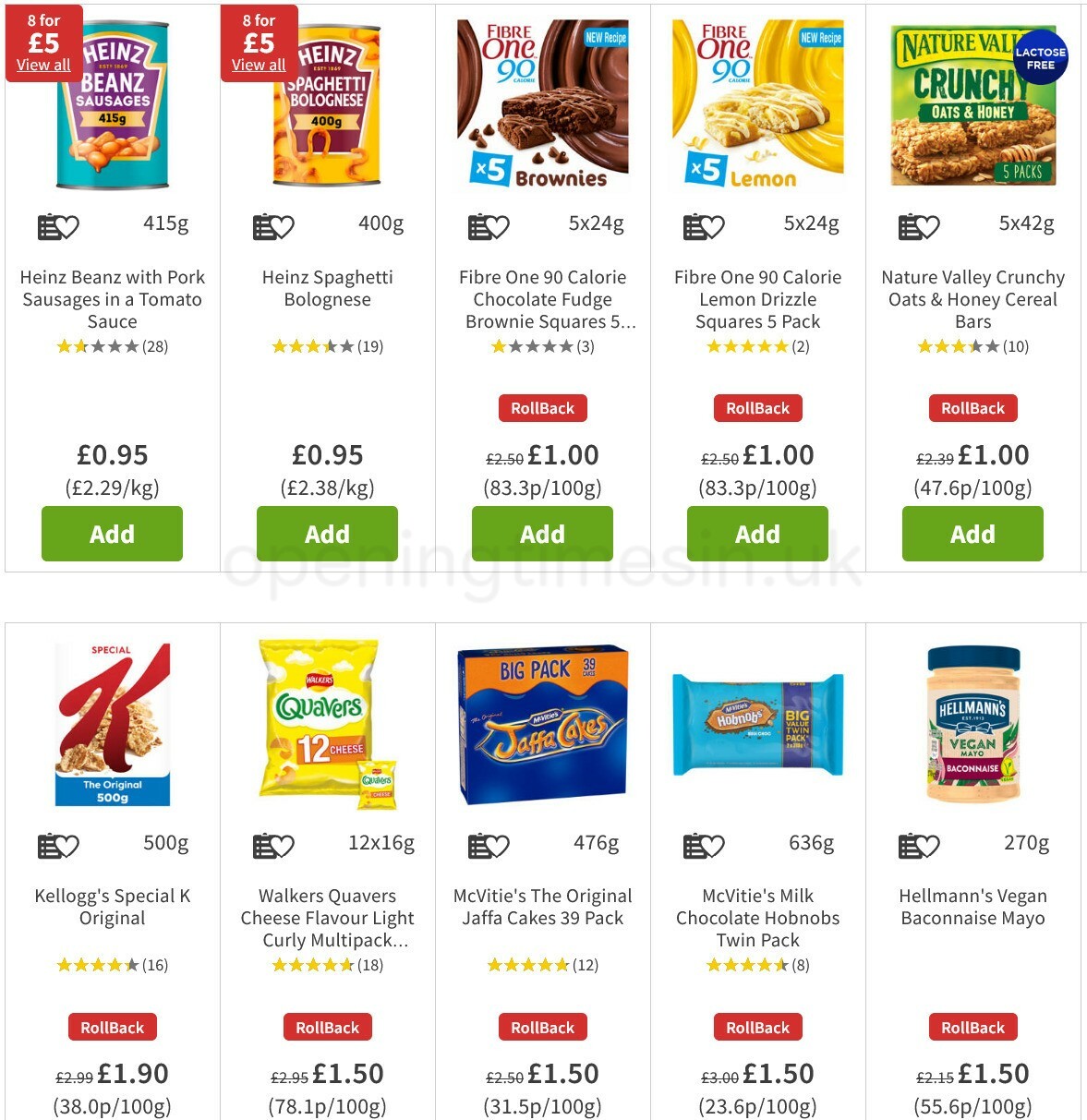Here's a cleaned-up and detailed caption for the image described:

The image features a white background showcasing 10 different products, each accompanied by stars and a heart, indicating user preference or popularity. At the top left, there is a red box containing Heinz Beans with Pork Sausages in Tomato Sauce, rated with 2 stars and highlighted as "8 for 5 euros." Next, adjacent is a white box with a red corner, offering Heinz Spaghetti Bolognese with a rating of approximately 3.25 stars, also priced at "8 for 5 euros."

Moving along, there are two Fiber One products, each marked with a blue "new recipe" label: a 5-pack of 90 calorie Chocolate Fudge Brownie Squares and a 5-pack of Lemon Drizzle Squares, both noted with hearts. 

Nature Valley Crunchy Oats and Honey Cereal Bars are presented next, featuring a lactose-free label and rated 3 out of 5 stars, with a heart symbol indicating popularity.

Below these, there is a Kellogg's Special K Original 500g box, highlighted as a rollback item priced at €1.90 and adorned with a red tag and a heart. Next, Walker's Quavers Cheese Flavored Light Curly Multi-Pack chips are presented with a rollback price of €1.50, marked by a heart.

Also featured are McVitie's Original Jaffa Cakes in a 39-pack with a perfect 5-star rating, and Milk Chocolate Hobnobs Twin Pack, rated 4.5 stars—both rollback priced at €1.50 and marked with hearts.

Finally, Hellman's Vegan Mayonnaise rounds out the selection, also priced at €1.50 with a heart symbol and indicated as a rollback item. Each product entry includes a green "Add" button at the bottom, inviting users to add the item to their cart.